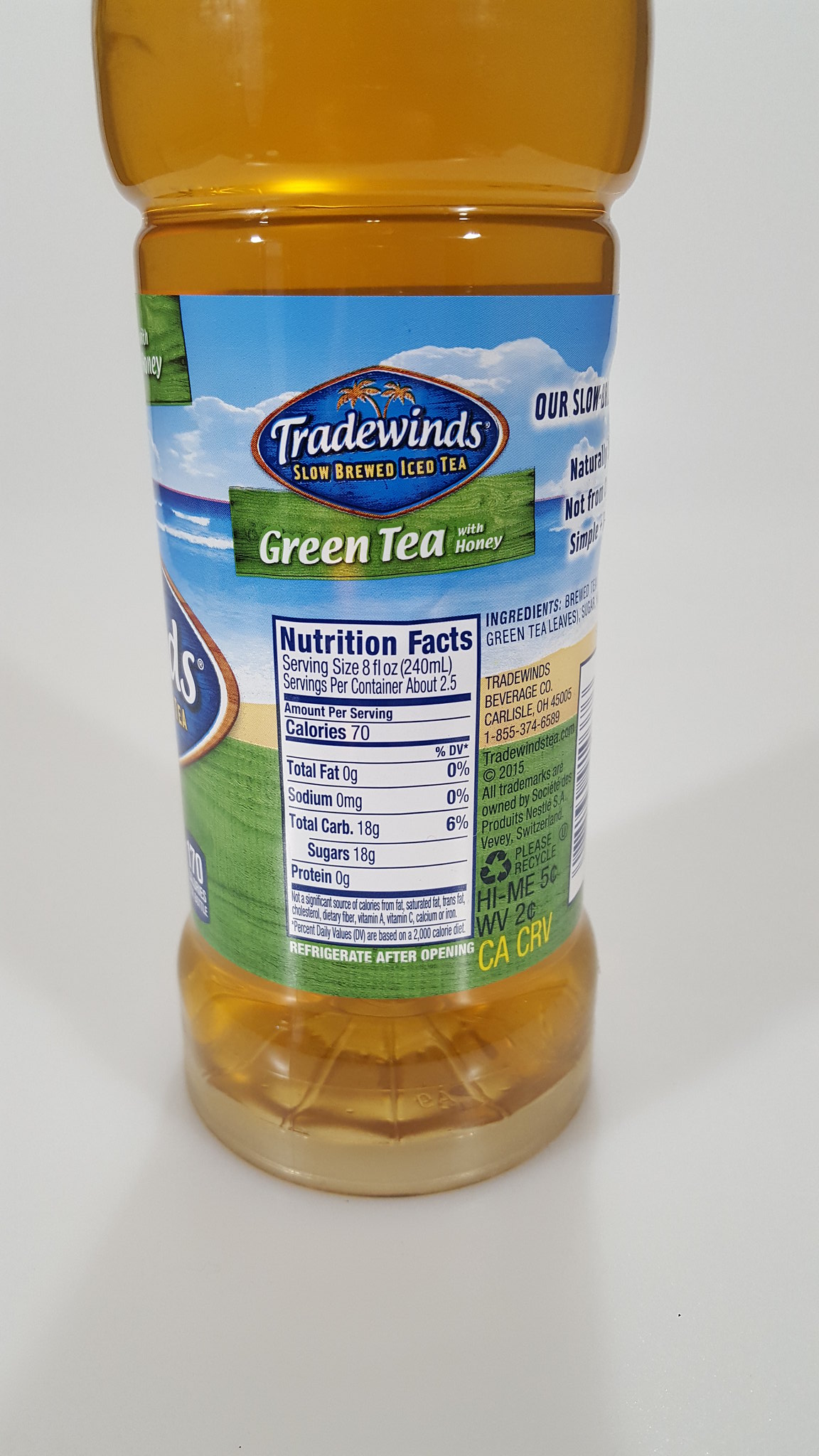This rectangular image, oriented vertically, features a bottle of iced tea prominently displayed against a pristine white background. The bottle rests on a matching white countertop, enhancing its visibility. Central to the composition is the bottle's label, which is captured in sharp focus.

The label showcases the brand "Tradewinds Slow Brew Iced Tea" with "Tradewinds" written in white text on a blue background. Below, "Slow Brew Iced Tea" is highlighted in a vibrant yellow. A green label beneath that reads "Green Tea with Honey" in crisp white lettering. Additionally, a white box bordered in black carries the "Nutrition Facts" in bold black text, providing detailed nutritional information.

The tea inside the bottle is a light brown hue, reminiscent of traditional iced tea or apple juice, emphasizing its refreshing quality.